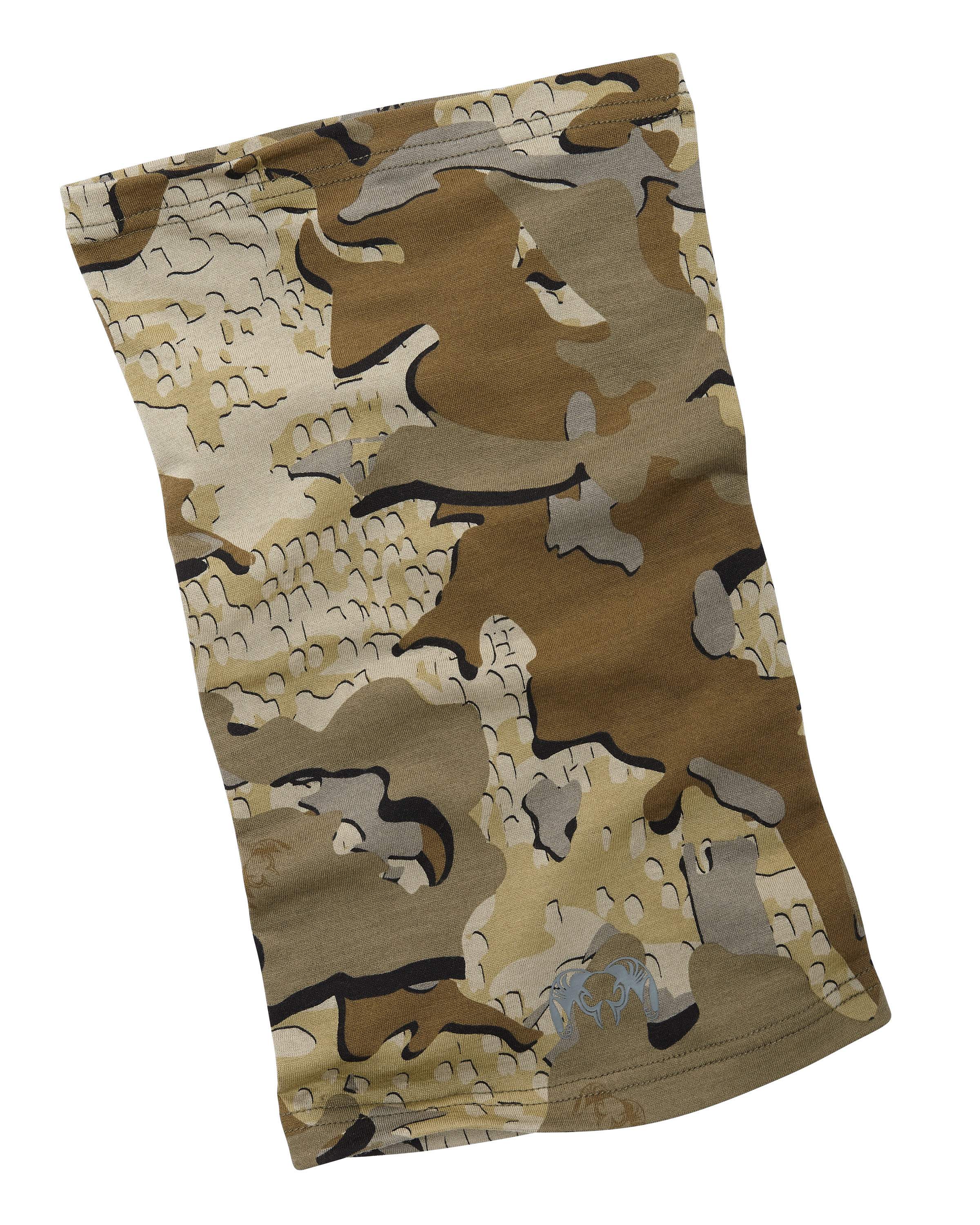This rectangular collage, oriented vertically, resembles a piece of fabric with visible stitching at the top and bottom edges. The collage appears to be composed of multiple layers, intricately cut away to reveal various shades of gray, green, and tan, interspersed with both lighter and darker grays. There are also small figures in light blue that add a dash of contrast to the overall composition. The entirety of the artwork is slightly tilted, creating a ripple effect akin to draped cloth, with noticeable shadows that give it a sense of depth and movement.